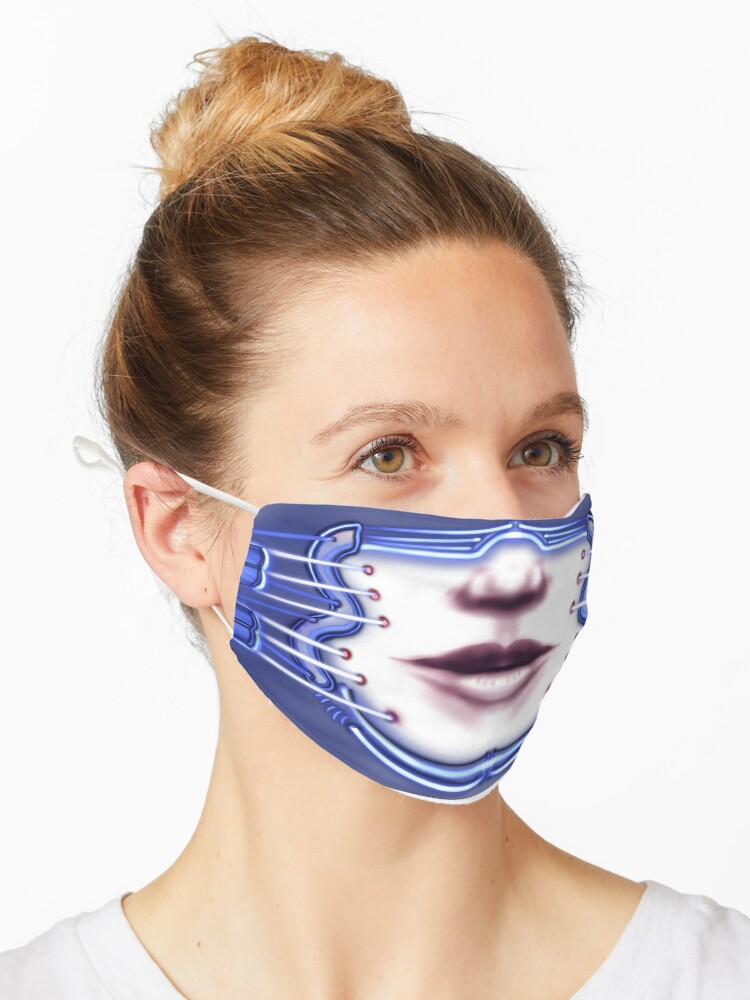In this close-up photograph, a model showcases a creative and humorous face mask against a completely white background. The focus is on the mask, which features a detailed design of a nose and mouth, creating a quirky optical illusion that makes it appear as if her mouth is open and unmasked. The model has light brown to dirty blonde hair, styled neatly into a bun, with the bun itself displaying a more blonde hue. Her striking hazel eyes vary between light brown and golden tones, adding depth to her expression. She is dressed in a white shirt, and a small, punctured hole for an earring is visible on her right ear, though no earring is present. Additionally, the strings of the mask are visible, extending from her cheek to the back of her ear, further emphasizing the realism of this playful mask design.